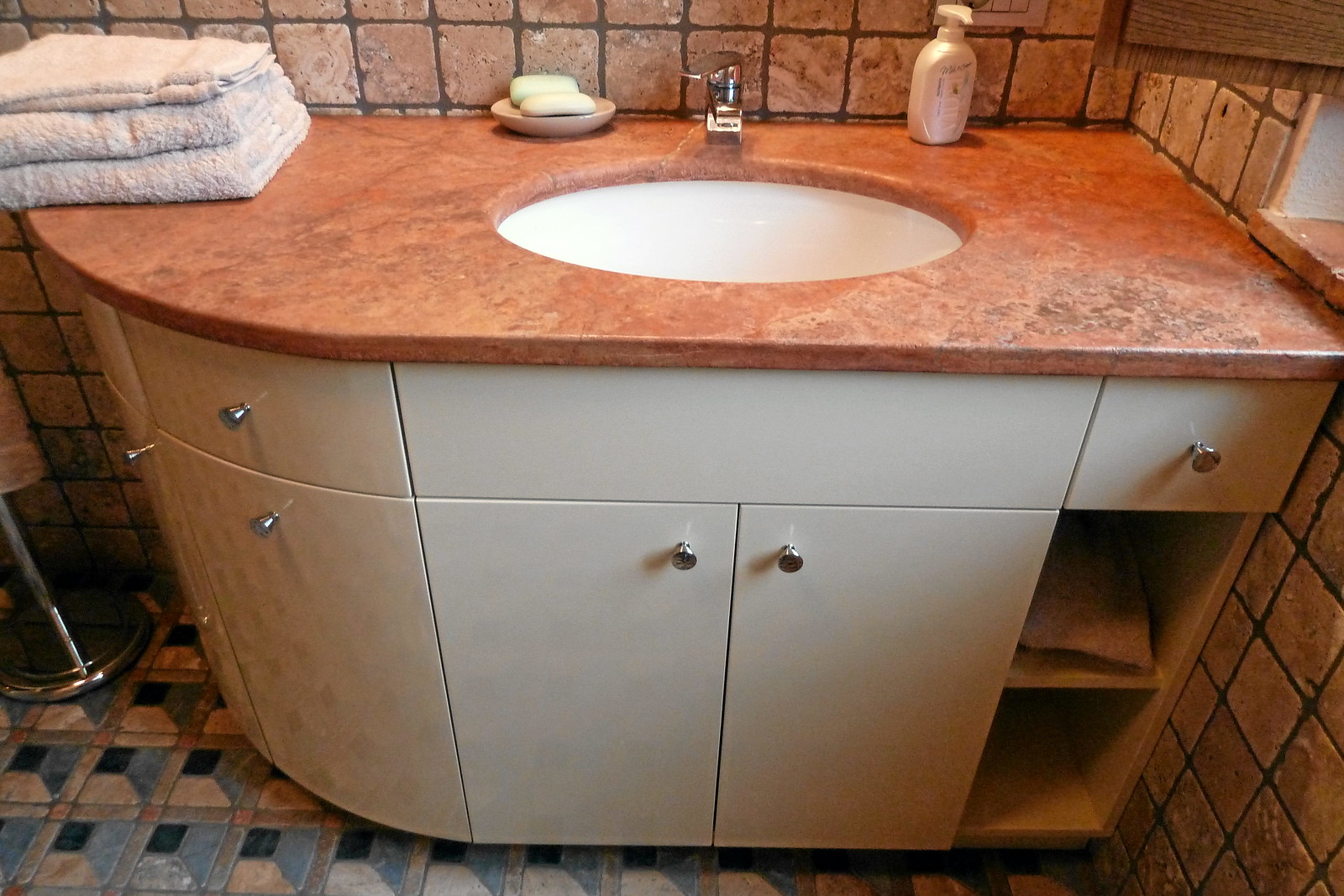The image showcases a close-up of a pristine white porcelain washbasin set into an elegant granite-look countertop. This countertop features a striking blend of orange and brown tones, perfectly complementing the bathroom's overall warm color palette. The walls are adorned with a stylish mix of light brown, dark brown, and cream-colored tiles, providing a rich, earthy backdrop. The floor contrasts beautifully with blue and brown square-patterned tiles. Beneath the countertop is a sleek, cream-colored cabinet sporting shiny silver knobs that add a touch of modern sophistication. Adding a practical yet decorative element, three neatly folded towels are placed in the left corner of the countertop, enhancing the bathroom's inviting and well-organized feel.